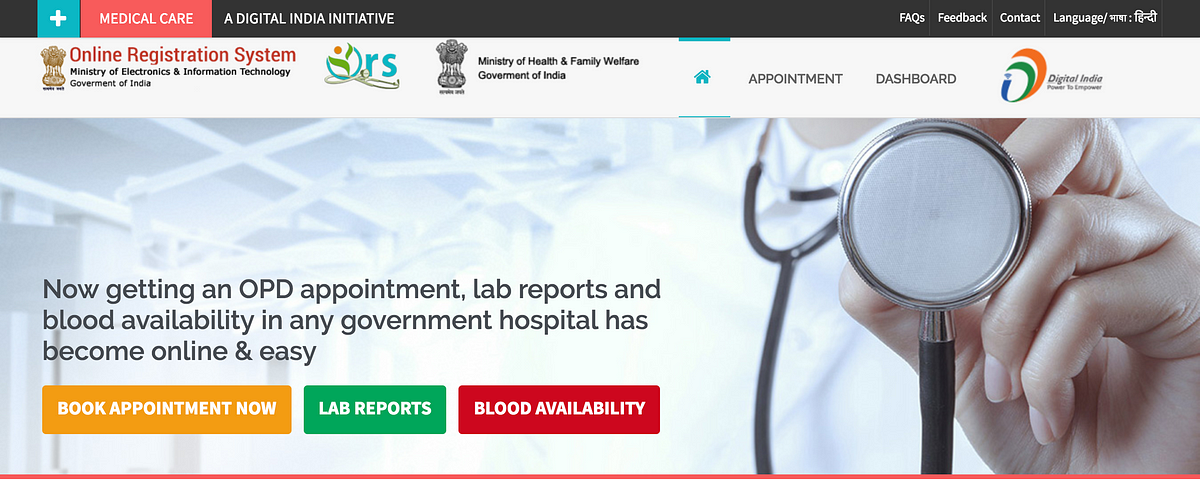The image depicts a healthcare website interface dedicated to online registration systems. Dominating the design is a black navigation bar extending across the top of the page, featuring menu options labeled "FAQs," "Feedback," "Contact," and an option related to "Language" settings.

Prominently displayed is a logo incorporating a green "D" resembling a flower and blue "R" and "S" characters. Beneath the logo is a tagline that reads, "Medical Care: A Digital India Initiative."

Below the tagline, a centrally-positioned photo features a doctor, likely a woman based on the visible hand size and neck, holding a stethoscope with her left hand. The stethoscope is prominently positioned in the center of the image, illustrating direct patient readiness. The background suggests the setting is a hospital, noticeable by the exposed beams and supports of an unfinished ceiling.

Accompanying the photo is a text box stating, "Now getting an OPD appointment, lab reports, and blood availability in any government hospital has become online and easy." 

Underneath this information are three distinct action buttons: 
1. An orange button labeled "Book Appointment Now."
2. A green button labeled "Lab Reports."
3. A red button labeled "Blood Availability."

These elements collectively emphasize the ease and accessibility of digital healthcare services provided through this online platform.